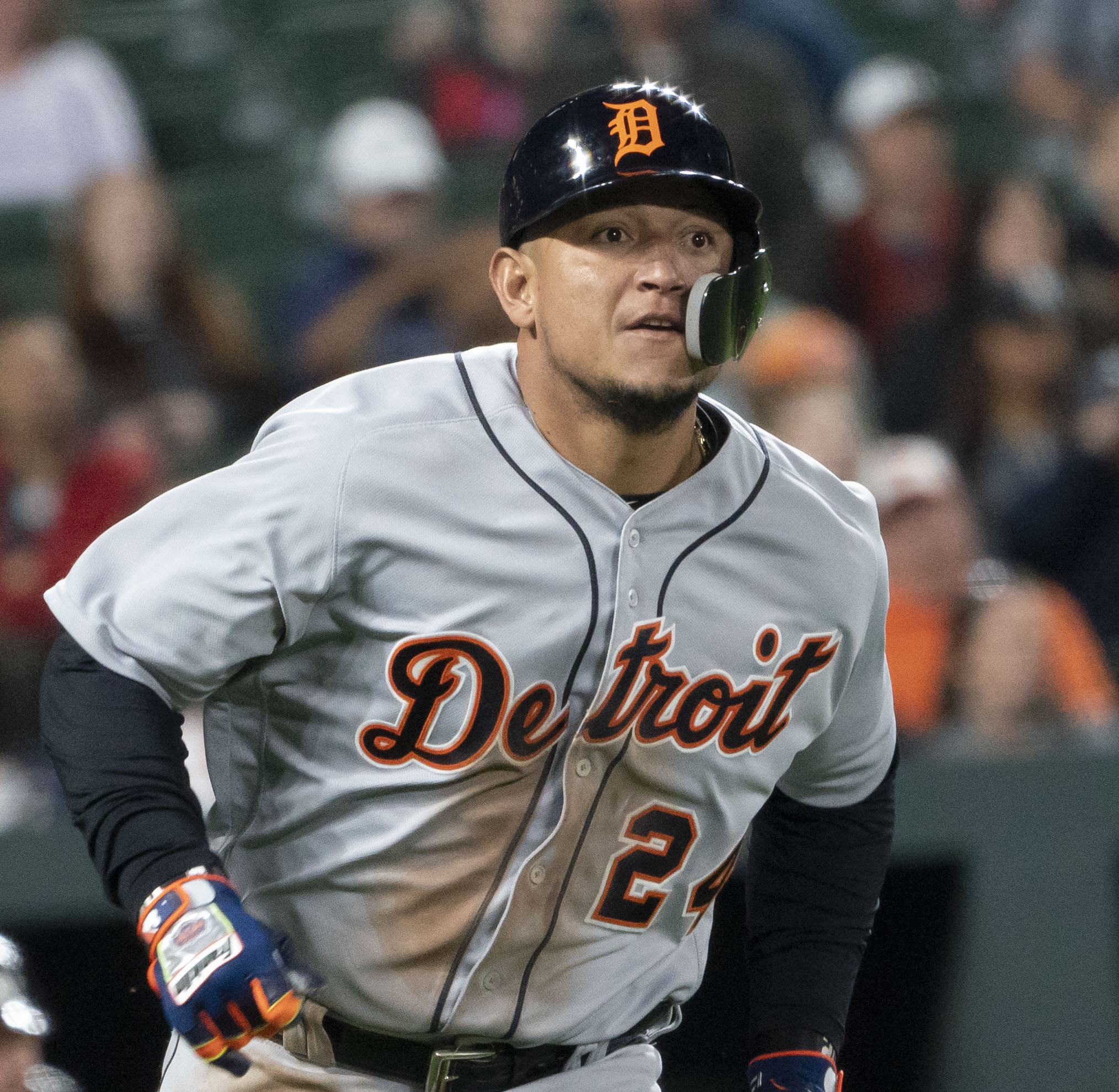This is a square photograph of a focused baseball player from the Detroit team. He's mid-action, appearing to look for a sign from the coach. The player is centrally positioned, surrounded by a blurred background of spectators in green seats, many of whom are wearing white ball caps. 

The athlete is clad in a gray, button-up jersey with "Detroit" boldly written across the chest in black and orange, edged with a white border. His uniform reveals the number 24, also bordered in white. He sports a black reflective helmet with an orange "D" on the front and a partial faceguard on the left side. 

Underneath his jersey, he wears a long-sleeved black t-shirt, and his hands are equipped with blue and orange Franklin batting gloves. His outfit is completed with gray pants fastened by a black leather belt with a silver buckle. The player’s eyes, which are distinctly brown, are slightly open and directed intently ahead, capturing a moment of focused anticipation. In the lower part of the image, a dark gray or black wall is visible just in front of the stands.